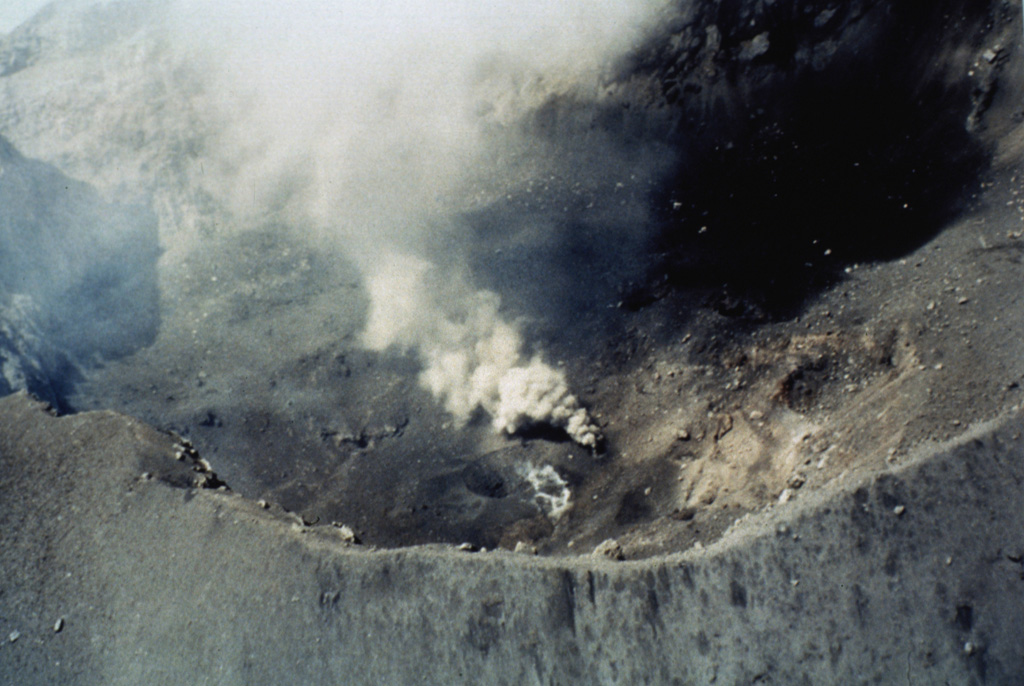This aerial photograph, possibly taken in the 1970s or 80s, depicts a tumultuous scene within the mouth of an active volcano. The image, though slightly grainy, offers a detailed look into the deep, crater-like pit characterized by dark, jagged rock formations in various shades of gray, brown, and black. The rocky surface appears fractured, with numerous fissures from which thick, grayish-white smoke billows upwards, suggesting imminent volcanic activity without any visible lava. The overall impression is one of a rugged, earthy landscape veiled in smoky plumes, evoking a sense of a volatile, otherworldly terrain.